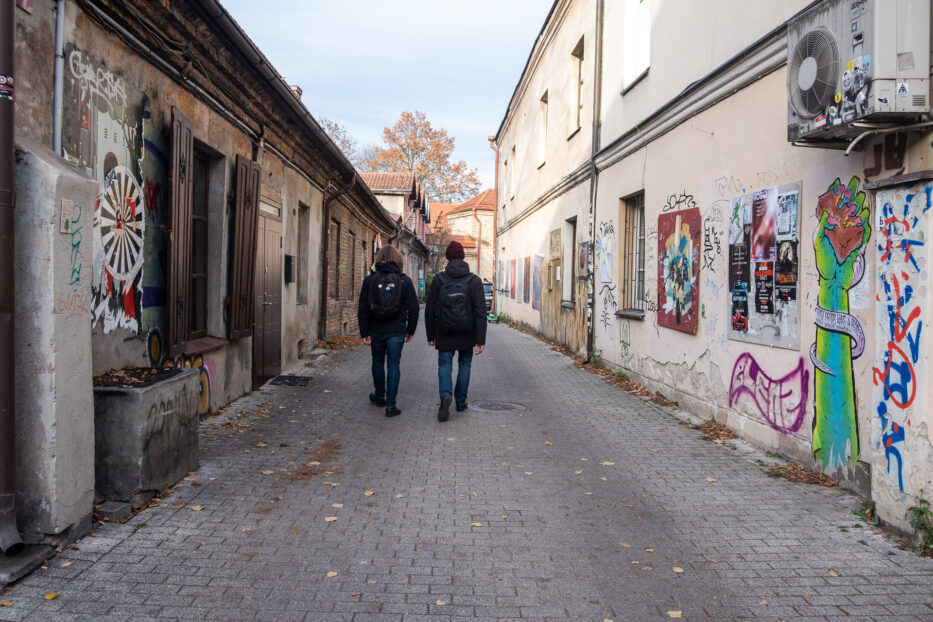In this photo taken outdoors in the middle of an alleyway flanked by buildings, two men are walking away from the camera. Both are wearing blue denim jeans, black jackets with hoods, black backpacks, and black shoes. The man on the left has long brown hair, while the one on the right sports a burgundy red beanie. The alleyway is paved with grey cobblestones or concrete.

On the left side of the alley, a one-story building with a flat roof houses brown wooden window shutters. Its brick or concrete walls are heavily graffitied, featuring a prominent black and white wheel with red markings. The building appears dirty and cluttered with debris like leaves.

The right side showcases a two-story beige building covered in extensive graffiti, making it look dilapidated with chipping paint. Highlighted on the wall is a vibrant piece of street art: a green and blue hand emerging from the ground, gripping something red, and wrapped in a purple snake tail. Additional graffiti includes blue and red letters and various frames.

The alley exudes a gritty urban atmosphere, artfully filled with street art and graffiti on both sides, creating a stark contrast with the pedestrian-only pathway between the buildings.